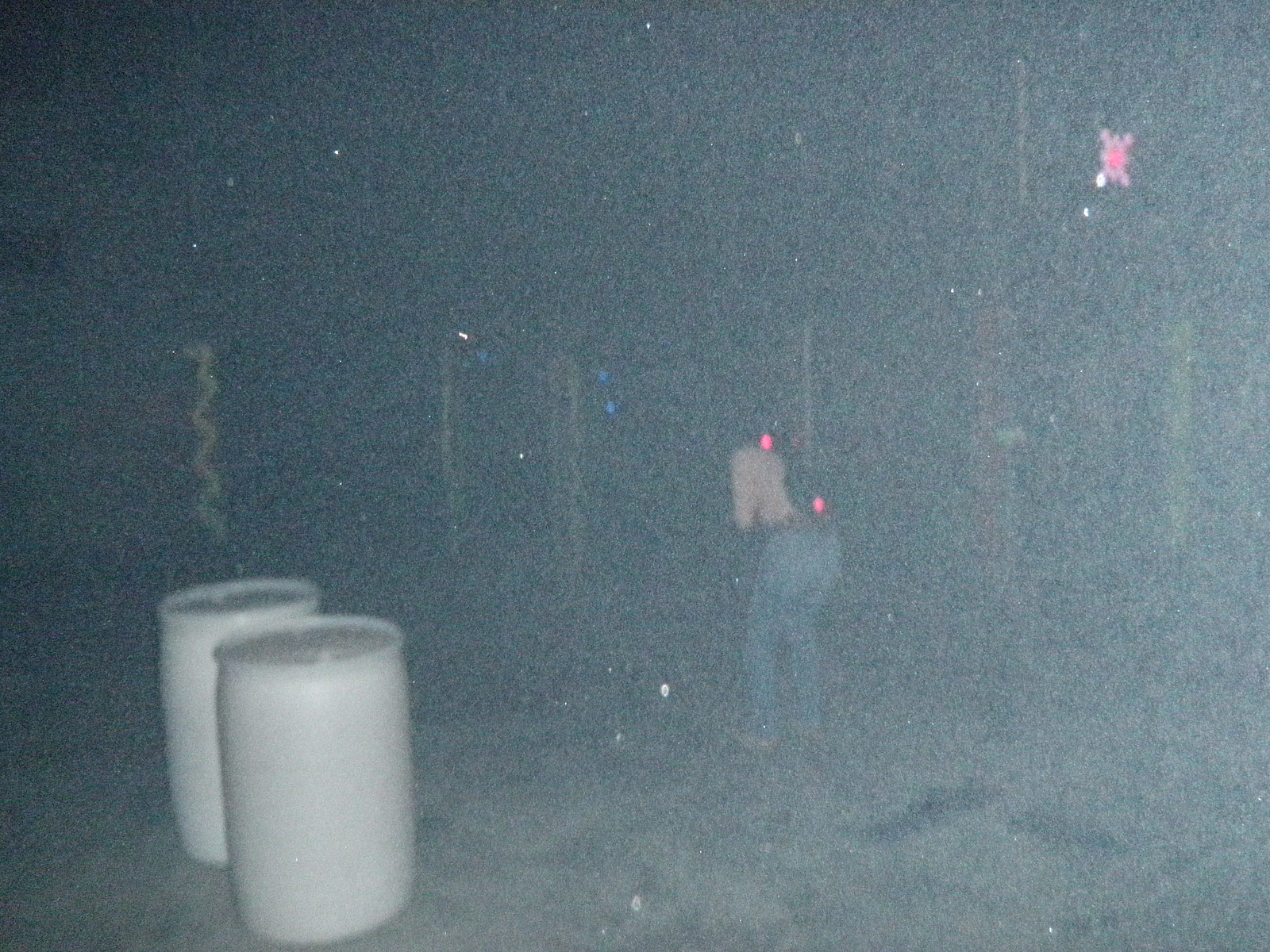The image is an extremely blurry and grainy photograph with various visual elements barely discernible. To the immediate left of the frame, there are two white 55-gallon plastic barrels with slightly raised rims, positioned one in front of the other. Centered in the photo, there appear to be two figures, one dressed in blue and another in a light or cream-colored top, suggesting a tan jacket or shirt. Notably, one of the persons seems to have parts of their back missing, potentially due to wearing a backpack. The figures are bathed in purplish light, possibly from a wearable source, and exhibit two red laser dot lights—one near the waist and another near the head. In the background, the image transitions into a very dark and hazy blue space, with hues of red and pink light, and a yellow squiggle above the barrels. The far right of the image features an indistinct purple object and hints of tree outlines or open clearance, amplifying the photo's overall blurry and obscure nature.